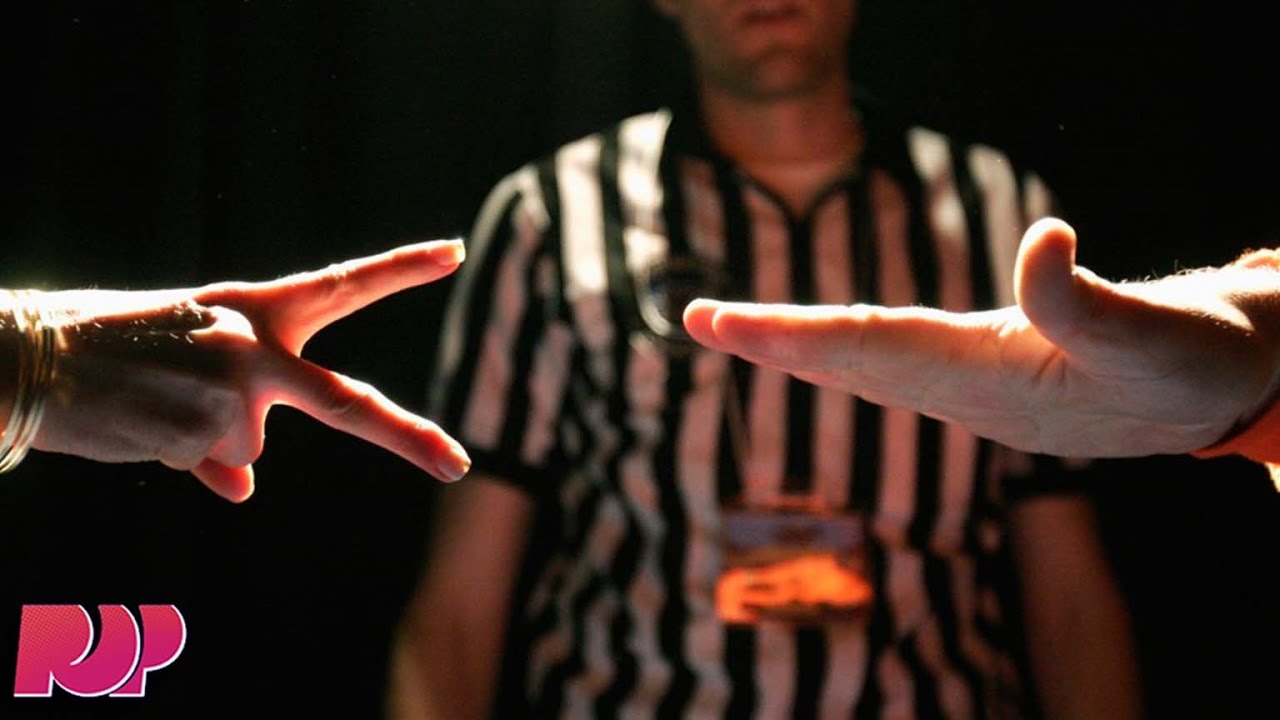This rectangular poster displays a photograph against a black backdrop, illustrating a game of rock, paper, scissors. On the left, a woman's hand, adorned with gold bracelets, is positioned in the scissors gesture, her fingers illuminated by a striking glare of light. To the right, a man’s hand, with light skin and a hint of a bright orange sleeve, is extended flat in the shape of paper, similarly highlighted by the light. Central to the image is a referee, clad in a black and white striped shirt, whose face is obscured except for his mouth. Around his neck hangs a lanyard with an amber-glowing tag or timer that rests just above his navel. The referee stands slightly out of focus, adding depth to the scene. In the bottom left corner of the poster, the bright pink letters "P.O.P" are prominently displayed.